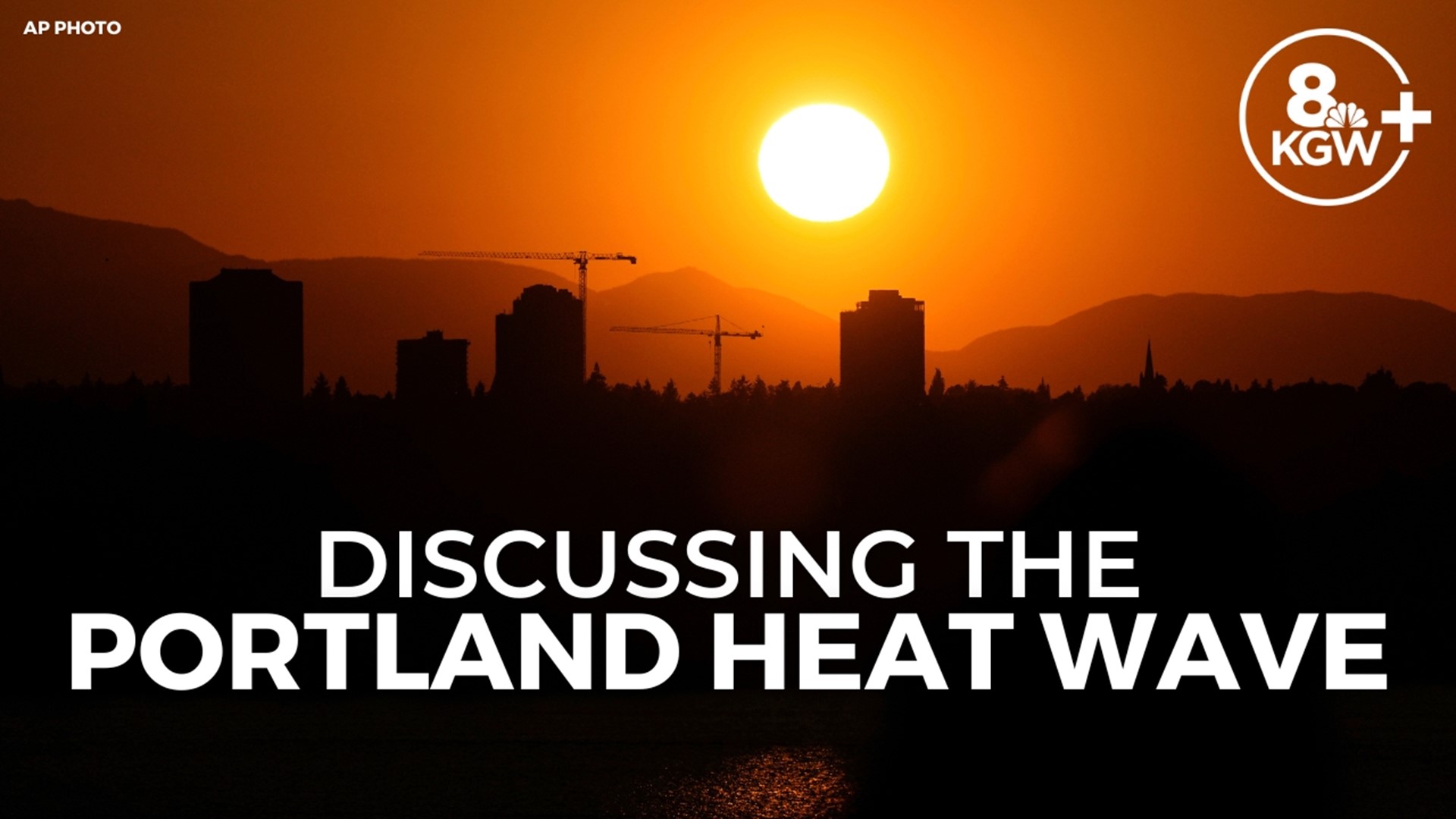This is a detailed photograph capturing a picturesque sunset over the Portland skyline. The image is framed in a rectangular shape, featuring a vivid color palette of bright yellow, deep oranges, and shades of brown. The sun, a radiant yellow ball, hovers just above a backdrop of silhouetted mountains, casting a warm orange glow across the sky. In the foreground, the skyline is depicted in dark browns and blacks, with distinguishable skyscrapers and tall construction cranes piercing the horizon. 

In the upper left corner, small white text reads "AP Photo," while the top right corner displays the logo for Channel 8, KGW, alongside the NBC peacock within a white circle, accompanied by a plus sign. Dominating the bottom part of the image in large, white font are the words "Discussing the Portland Heat Wave," indicating this commercial still is likely from a news segment discussing the local weather phenomenon. The lower part of the image remains black, obscuring additional details below the skyline. The photograph exudes a striking contrast between the illuminated sky and the shadowed cityscape, artistically capturing a significant moment in time.